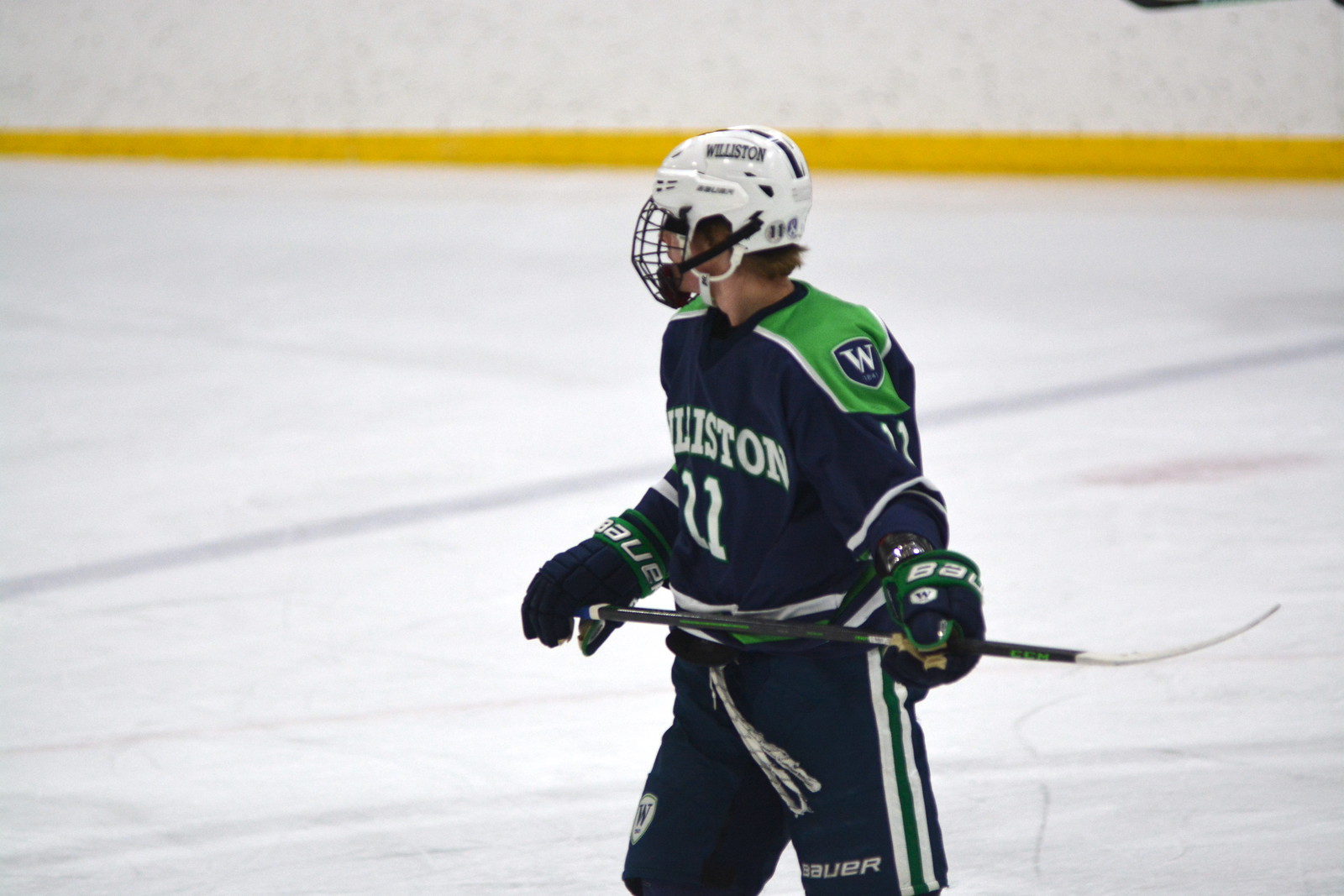The image captures a teenage hockey player on the ice, set against a backdrop of the rink. The majority of the background, about 80% up the image, consists of the ice, marked with various lines typical of a hockey rink. There's a yellow bar running horizontally across the top of the ice, separating it from a blank white wall, indicating that the scene is not of a large arena but a more modest setting. The main subject in the foreground is dressed in a blue uniform with white writing and features a green section on the shoulder, trimmed with white near the green area and at the bottom of the waist. His gloves match his blue outfit and are detailed with green trim, while his pants are blue with white and green stripes along the sides. The player, identifiable as number 11, has the name "Williston" on his white helmet and "Liston" partially visible on his jersey. He is holding a black hockey stick with white tape on the blade, positioned in a padded block stance with his torso oriented slightly to the left and his head turned even more to the right. Additionally, there's a shield logo patch on his shoulder featuring a "W" and what appears to be "1841." The background simply shows the ice, reinforcing the focus on the player.